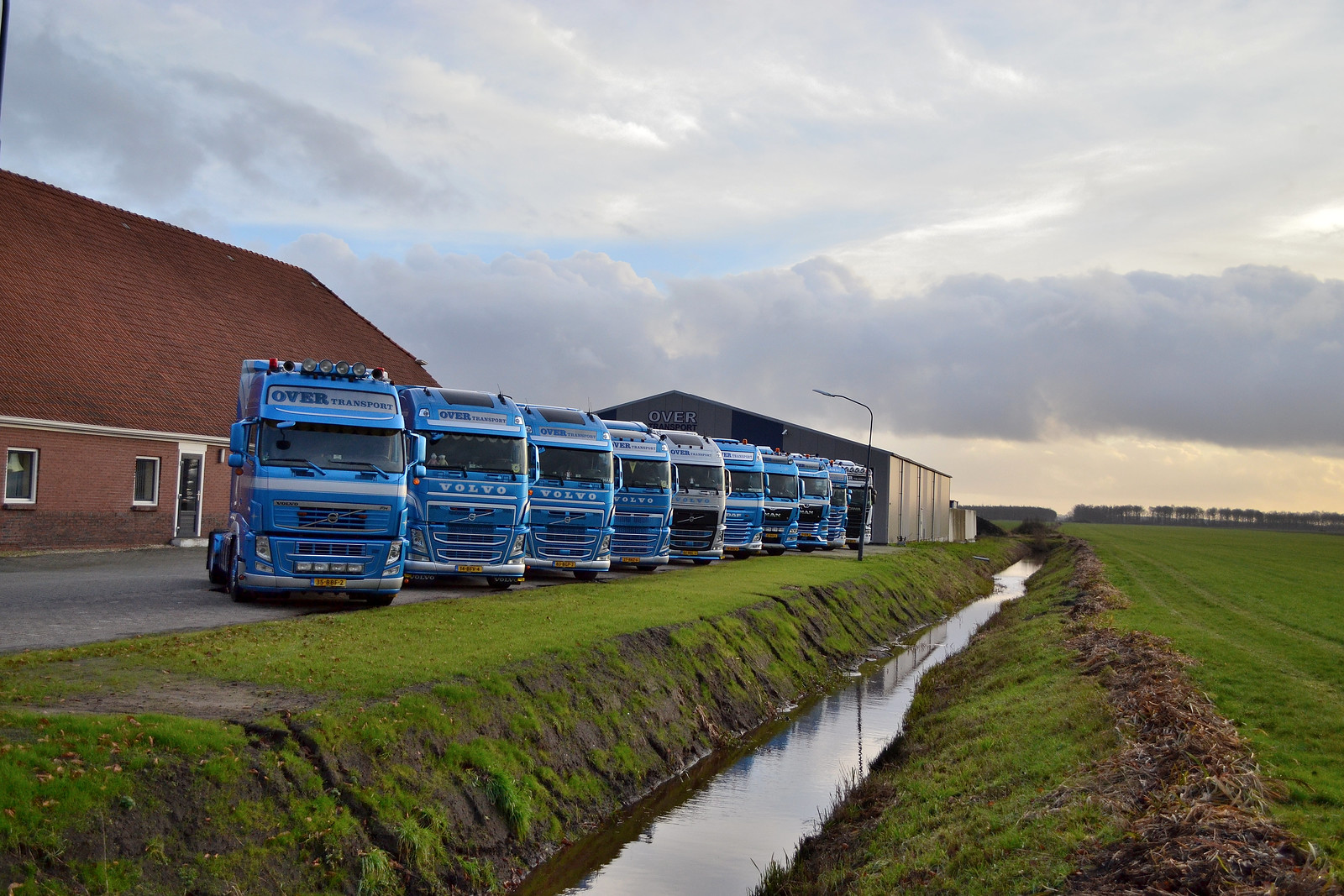In this outdoor scene, the sky is mostly filled with gray clouds, though some blue patches are visible. Dominating the foreground is a brick building with a reddish-brown sloped roof. Adjacent to this structure, a series of seven or eight blue Volvo trucks, each lacking the trailer, are arranged in a parking area, with their tops displaying the inscription "OVER transport" or "OVER Keenport." Among the blue trucks are a couple of gray ones, standing out slightly against their uniform backdrop. 

To the right of the brick building is a smaller gray shed with the word "OVER" marked on it. In front of the trucks stretches a grassy area, interrupted by a canal filled with water, which gives way to an expansive field of green grass. This field extends up to a distinctive tree line in the background. The setting appears to be either early in the morning or late in the evening, offering a calm and almost pastoral atmosphere reminiscent of a flat landscape, possibly akin to those in the Netherlands.